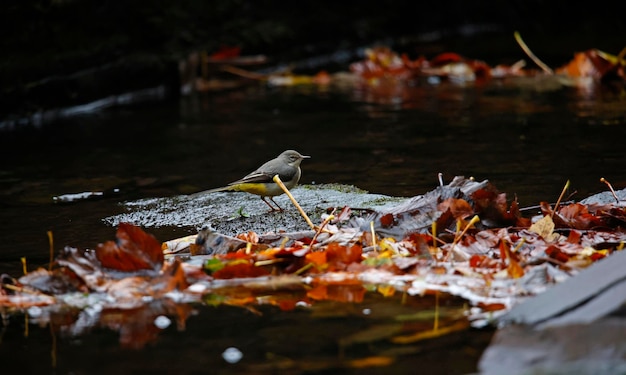This color photograph, in landscape mode, captures a serene autumn scene with a rich, dark color scheme. The focus is on a small gray bird with a hint of white on its tail, perched slightly left of center on a piece of wood. Surrounding the bird are vibrant red, yellow, and orange autumn leaves, some floating and some settled deeply in the dark, murky water, indicating a creek or riverbed. The background fades into near-black, enhancing the autumnal hues and the serene, contemplative mood. The bird, the only animal present, faces right, seemingly lost in thought. Additionally, tiny bubbles in the water suggest subtle movement, further enriching the scene's tranquil atmosphere.